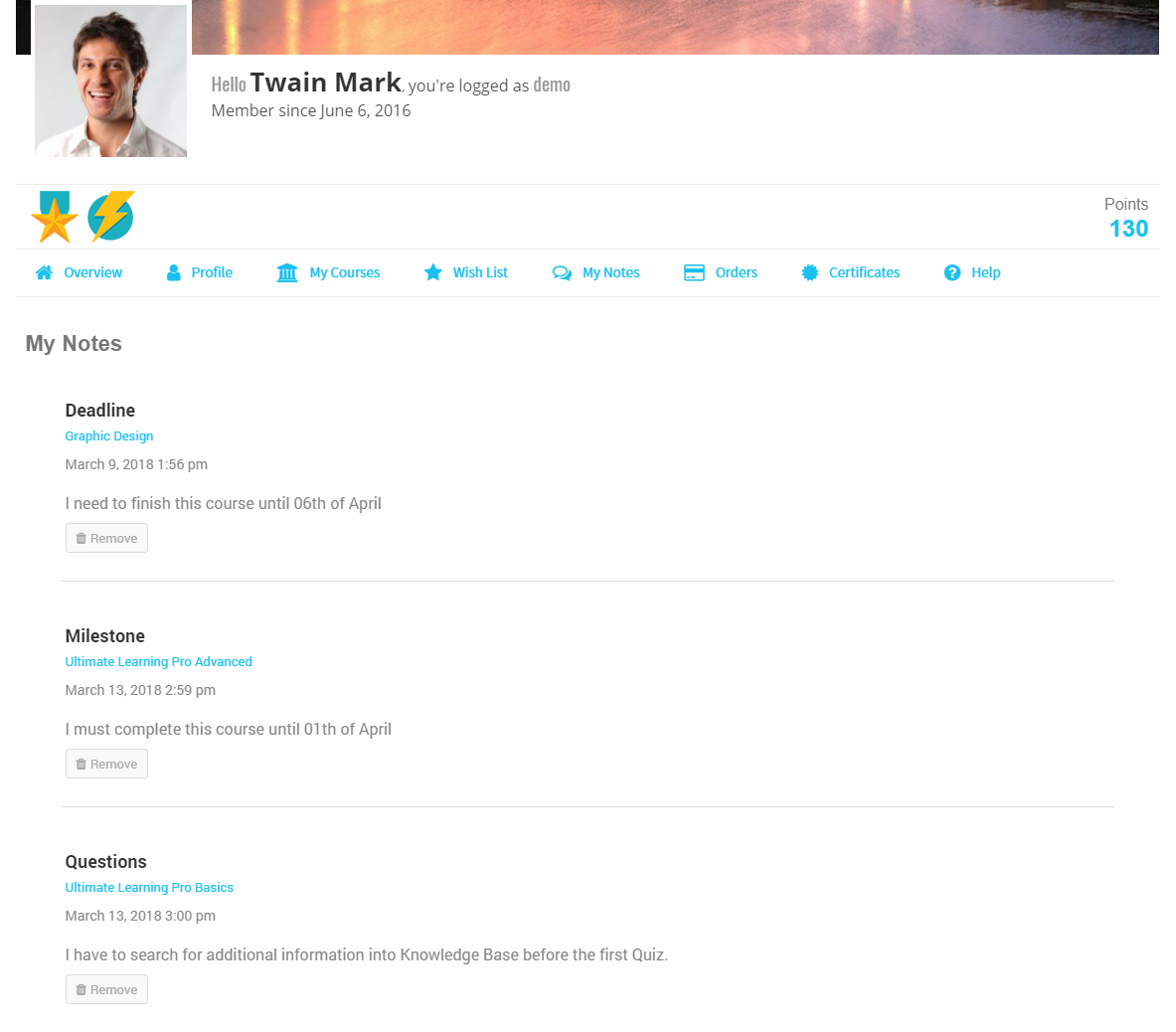The webpage appears to be a personal dashboard for a user named Twain Mark, who is identified as a demo member since June 6, 2016. On the left side of the screen, there's a photo of a smiling man. To the right, there's a welcome message that reads, "Hello Twain Mark, you're logged in as demo member since June 6, 2016."

Below this greeting, there is a medal icon featuring a star and a lightning bolt within a circle, both in green. The page includes various tabs for navigation: Overview, Profile, My Courses, Wishlist, My Notes, Orders, Certificates, and Help. Twain Mark has accumulated a total of 130 points.

Under the "My Notes" section, there are several entries:
1. **Deadline:** For the "Graphic Design" course, with a deadline marked as March 9, 2018, 1:56 PM. There's a note indicating the need to finish this course by April 6. There are options to remove this note, indicated by a trash can and remove button.
   
2. **Milestone:** For the "Ultimate Learning Pro Advanced" course, noted on March 13, 2018, at 2:59 PM, stating that it must be completed by April 1. Similarly, there are options to remove this milestone.
   
3. **Questions:** For the "Ultimate Learning Pro Basics" course, dated March 13, 2018, at 3:00 PM. The user is reminded to search for additional information on technology before the first quiz. This note also includes the remove options.

Overall, the webpage serves as a comprehensive dashboard providing Twain Mark with essential details regarding his learning progress and upcoming deadlines.